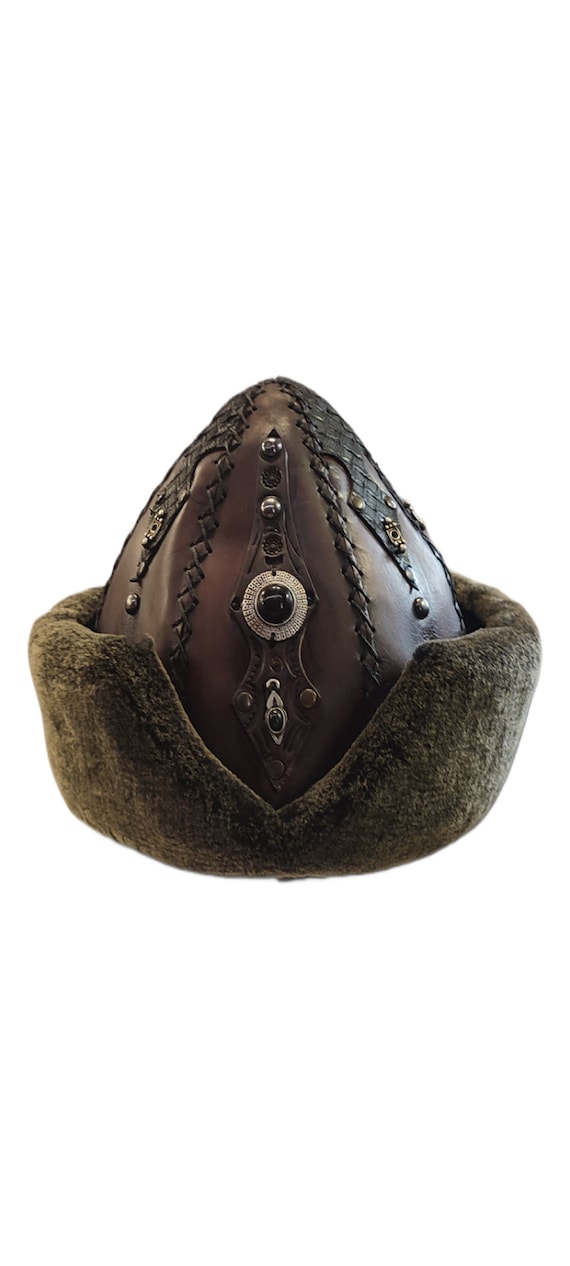This photograph features a unique, antique-looking hat crafted from brown leather. The hat has a conical shape, coming to a point at the top, with intricate leatherwork and stitching that runs up its seams, indicating it is assembled from multiple pieces of leather. The front of the hat is adorned with a prominent silver medallion set with a black stone, accompanied by two smaller silver pieces above and one below. Additional sections of the leather feature decorative stamp work and metal tabs, enhancing its ornate appearance.

Around the base of the hat is a fur collar that is turned up all the way around, resembling an egg sitting in a moat. The fur collar, which provides an intriguing contrast to the structured leather top, is split at the center and rises about a third of the way up the hat, enhancing its medieval or cultural aesthetic. This distinctive piece, with its blend of leather, silver embellishments, and fur, appears to be both a functional winter cap and a highly ornate, historical accessory.